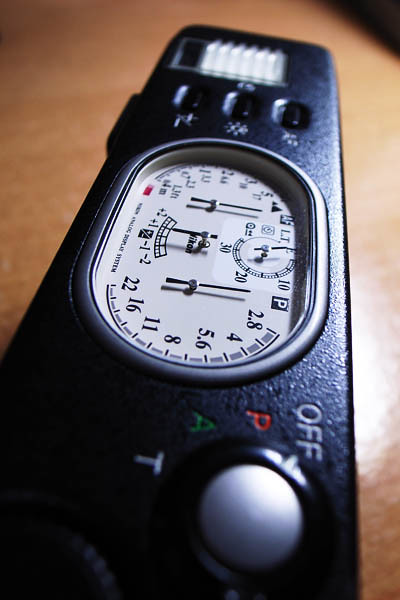In this image, there is an object positioned diagonally from the bottom left towards the upper right, though it doesn’t reach the upper right corner. The object is placed on a light brown wooden table, which fills the entire background except for a small dark triangular section in the top right corner, extending about 5% diagonally downward. The table’s surface reflects light, particularly striking at the bottom right of the image.

The object in focus appears to be turned to its side, revealing several details. On the bottom right of the object, the word "OFF" is written in white text. Below this, there are three letters: a red "P," a green "A," and a white "T." At the center of the object, there is a small display featuring a number system against a white background. The numbers listed are 2.8, 4, 5.6, 8, 11, 16, and 22, located towards the bottom middle of the object. Additionally, the top part of the object, positioned near the middle of the image, contains three black buttons.